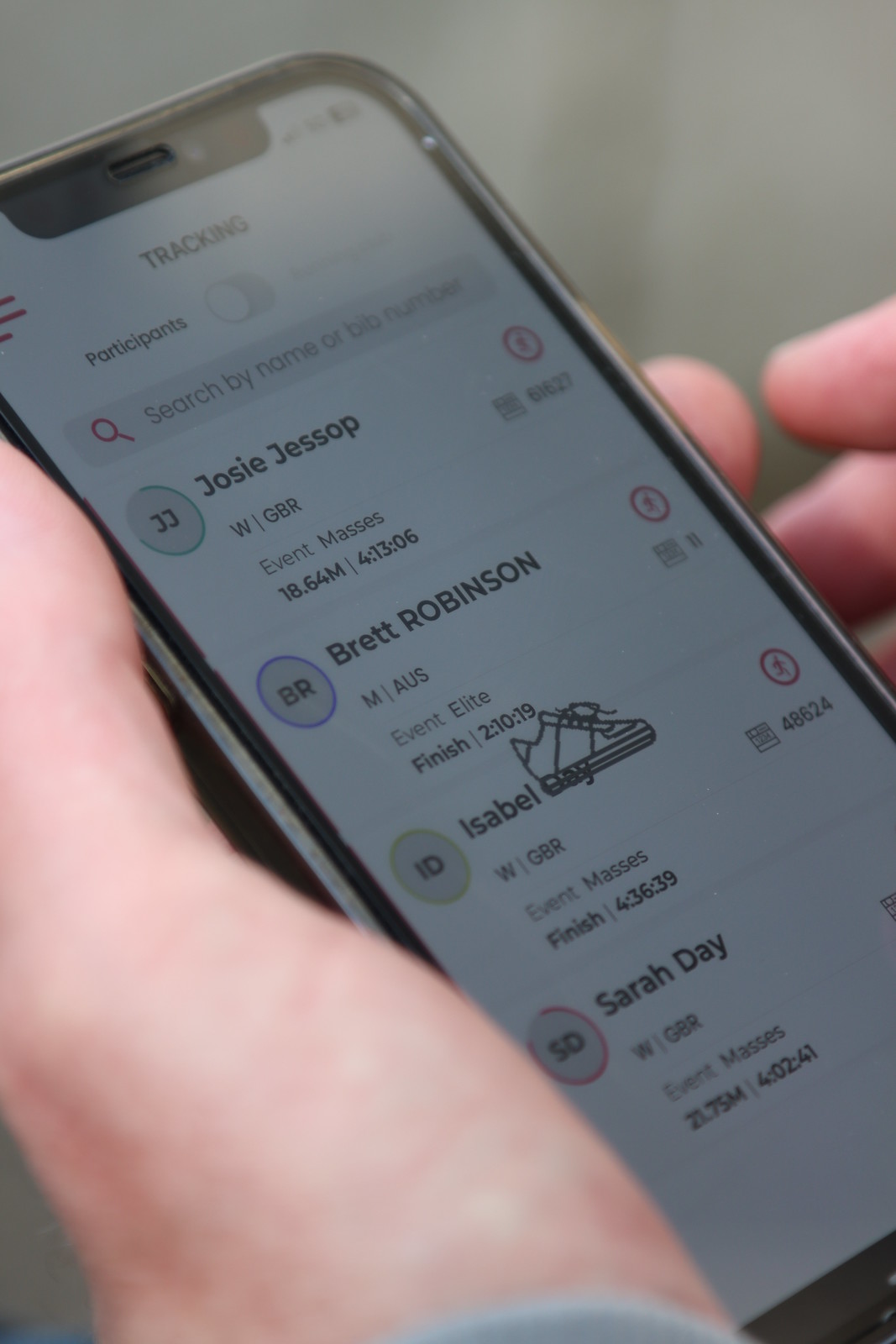The image shows an individual holding an iPhone with a tracking app open on the screen. The app displays the tracking statuses of several participants in a race. At the top, it shows the title "Tracking" and lists participants alongside their event names and times. The participants include Josie Jessup, with an event mass of 18.64 m for 1306, and Brett Robinson, who has an event finish time marked as elite at 210.19. Another participant, Isabel, whose last name is partially obscured by an animated shoe icon, has an event mass finish time listed as 436.39. The final name visible is Sarah Day, with an event time of 21.75 and a mass finish time of 4.02.41. The central shoe icon reinforces the context, indicating that the app is used to track these individuals as they participate in a race.